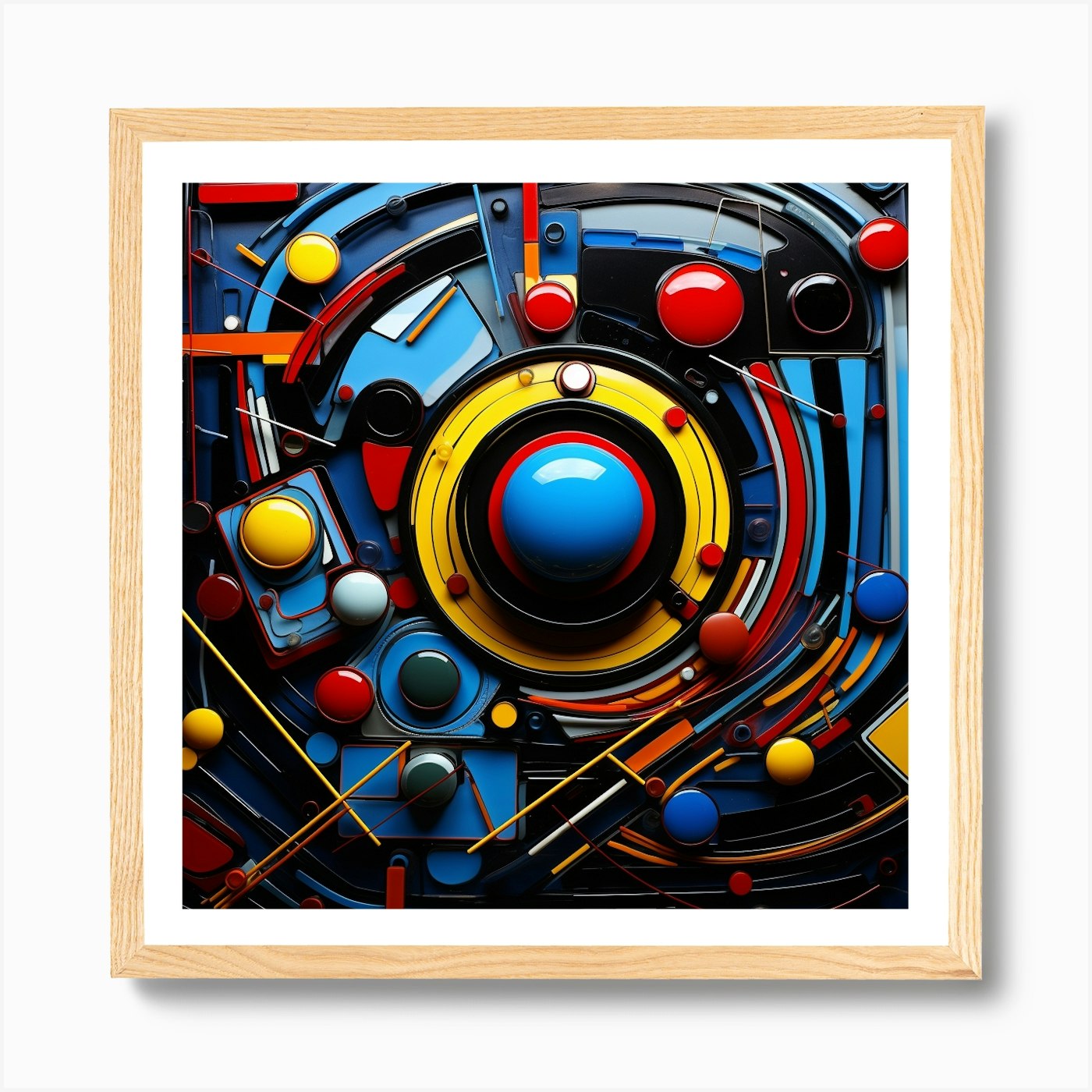The image features an abstract artwork encased in a square wooden frame with a white inner border. The artwork comprises a series of buttons in various bright colors, prominently including red, yellow, black, light blue, white, and green. In the center, a large light blue button is surrounded by concentric circles of red, black, and yellow. Additionally, the piece is adorned with scattered blue and orange geometric shapes, resembling sticks or lines, placed haphazardly across the white background. The buttons and geometric forms have a glossy finish, lending a tactile appearance to the arrangement. A soft drop shadow to the right side enhances the dimensionality of the painting, although there is no text to provide further context. The playful composition evokes a sense of randomness and abstract creativity.